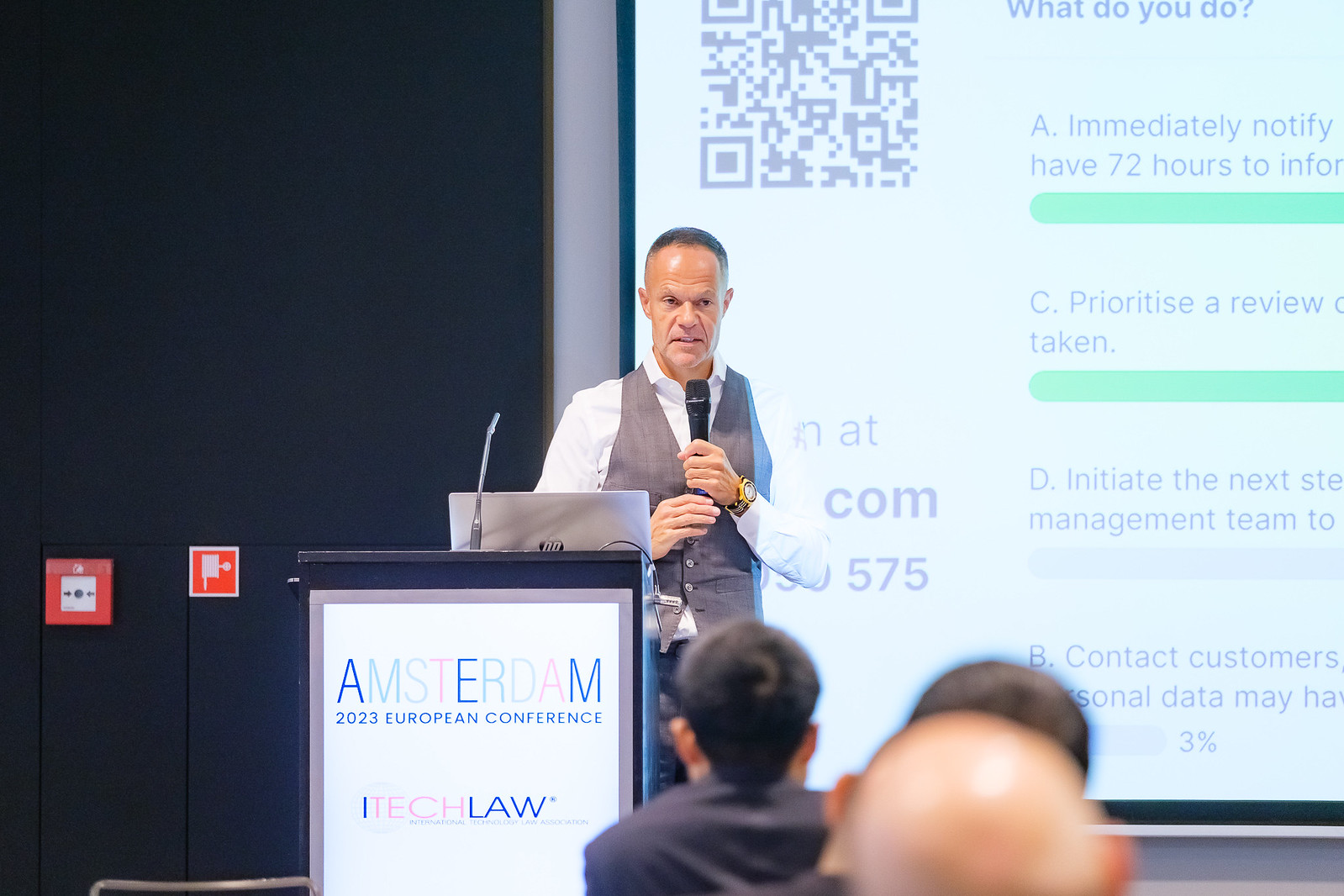In the photograph, a middle-aged Caucasian man with a receding hairline and salt-and-pepper hair stands on stage behind a podium, delivering a presentation at the 2023 European Conference in Amsterdam. He is dressed in a white dress shirt under a gray vest and sports a flashy gold watch. The podium displays a sign that reads "Amsterdam 2023 European Conference" and "Tech Law" alongside a relevant logo. The man holds a microphone and has an open HP laptop in front of him. Behind him, a large illuminated screen shows part of his presentation, including a multiple-choice question with options labeled A, C, D, and B and meters indicating audience responses. The text at the top of the screen reads, "What do you do?" The setting is a dark hall with a black wall, and in the foreground, the backs of three audience members' heads, including a bald man, are visible.